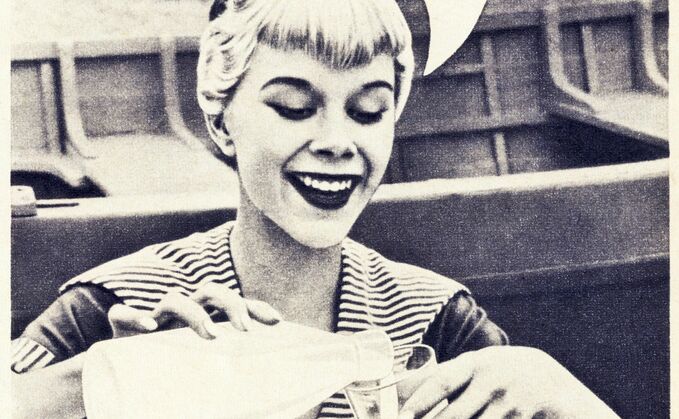In this vintage black-and-white photograph, a woman with short blonde hair, possibly styled in a bun (though it’s cut off at the top of the image), is captured mid-action as she pours herself a glass of milk. She is dressed in a classic sailor's outfit, complete with a prominent black-and-white striped collar that evokes the nautical attire of yesteryears. A hint of a sailor's hat suggests its presence on her head, visible on the right edge of the frame. The setting appears to be near a wooden rowboat. The woman is smiling warmly, her eyes focused down on the glass as she pours, and her expression is enhanced by visible eye makeup and lipstick. Her genuine smile, revealing her teeth, adds a lively character to this charming scene.